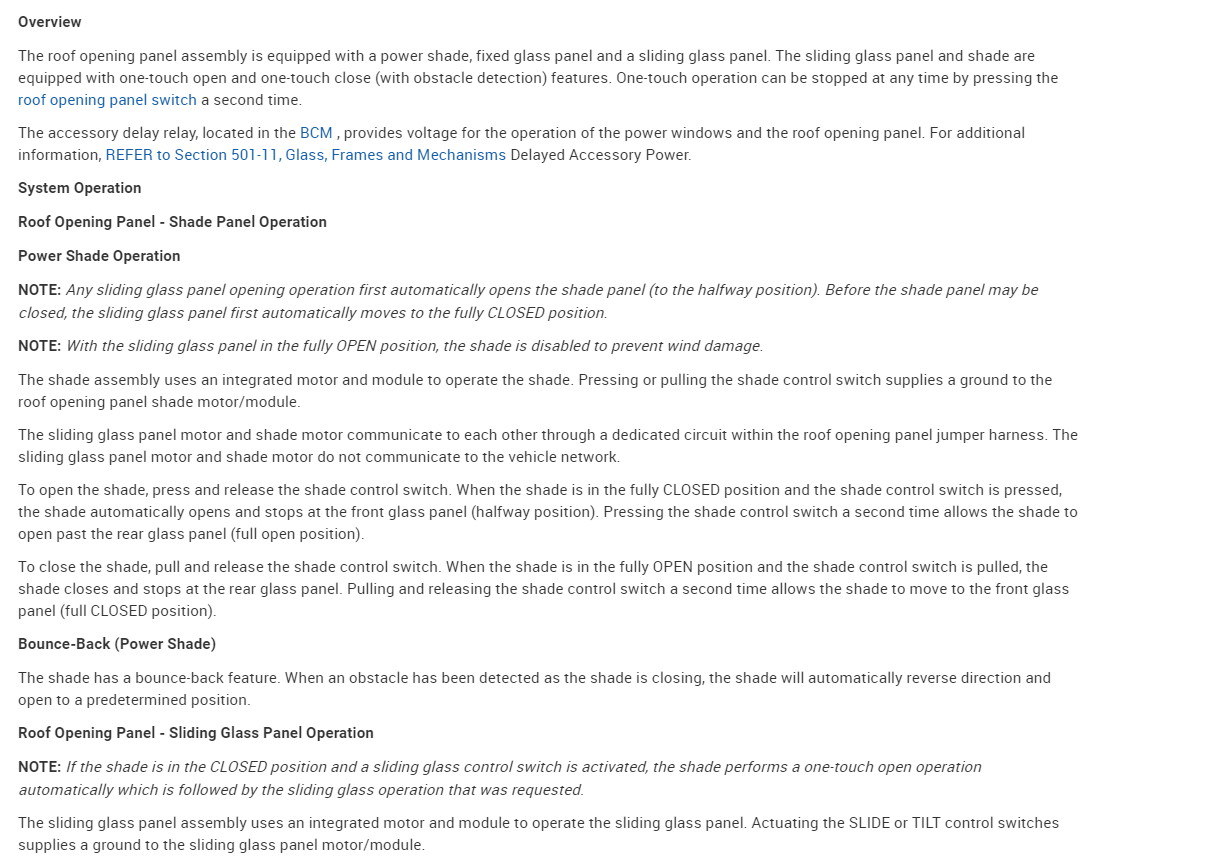This image is a screenshot of a web page featuring detailed technical specifications and operation instructions for a roof opening panel assembly. The webpage is characterized by a white background densely filled with text. 

The highlighted content describes a roof opening panel assembly that includes a power shade, fixed glass panel, and sliding glass panel. Both the sliding glass panel and the power shade offer one-touch open and close functionalities, complete with obstacle detection features. The one-touch operation can be interrupted by pressing the roof opening panel switch again.

An accessory delay relay in the Body Control Module (BCM) supplies the necessary voltage for operating the power windows within the roof opening panel. Additional details can be found in Section 501.11, which covers Glass Frames and Mechanisms and Delayed Accessory Power systems.

The system's operation specifics are outlined as follows: any operation to open the sliding glass panel automatically moves the shade panel to the halfway mark. Closing the shade panel requires the sliding glass panel to first close completely. To prevent wind damage, the shade is disabled when the sliding glass panel is fully open.

The shade assembly utilizes an integrated motor and module for operation. Activating the shade control switch links to the roof opening panel's shade motor/module. Notably, the sliding glass panel motor and the shade motor communicate via a dedicated circuit within the roof opening panel jumper harness, but they do not interface with the vehicle's network.